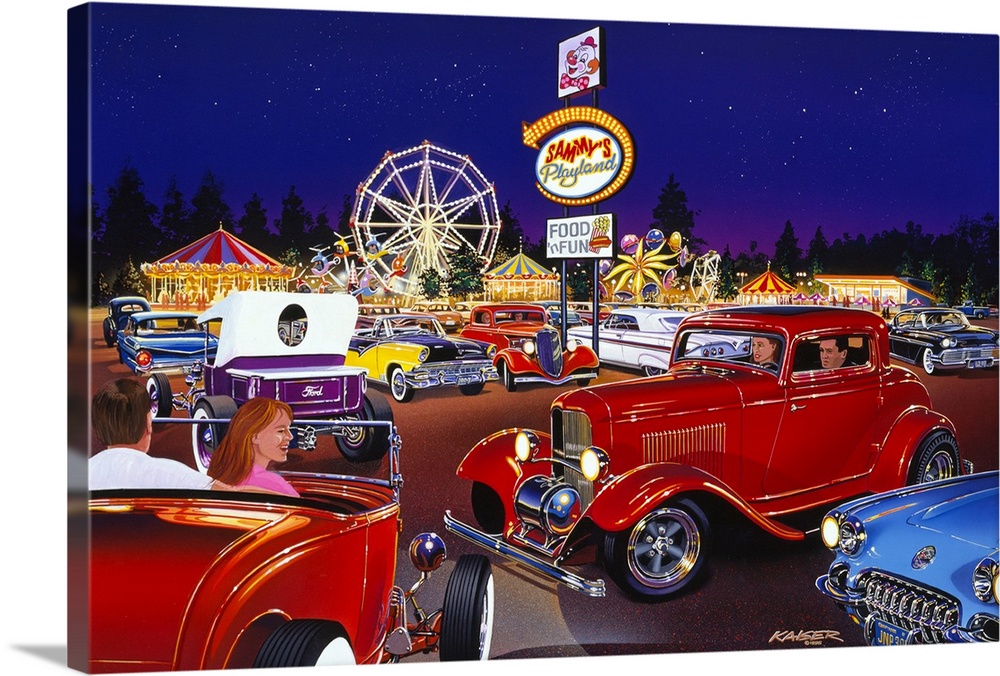The painting on the canvas depicts a nostalgic, retro scene of an old amusement park called Sammy's Playland, set against a starry night backdrop. The foreground features a bustling parking lot filled with colorful 1950s-1960s cars, including vibrant reds, deep blues, a striking purple, black, and yellow vehicles. Noteworthy are two red cars in the very front; one is a hot rod convertible with a man and a red-haired woman smiling beside him, while another red car shows a couple, seemingly waiting in line. At the center of the scene stands an illuminated sign with a clown on top, boldly reading "Sammy's Playland" and boasting "Food and Fun" with images of popcorn and a hot dog. Just behind the sign lies the heart of the amusement park, which features a central Ferris wheel, a helicopter ride, and a carousel, surrounded by other rides and a ticket booth with purple umbrellas. Adding depth, the playland and parking lot are framed by shadowy trees, capturing the lively yet serene atmosphere of a classic, nighttime fairground.